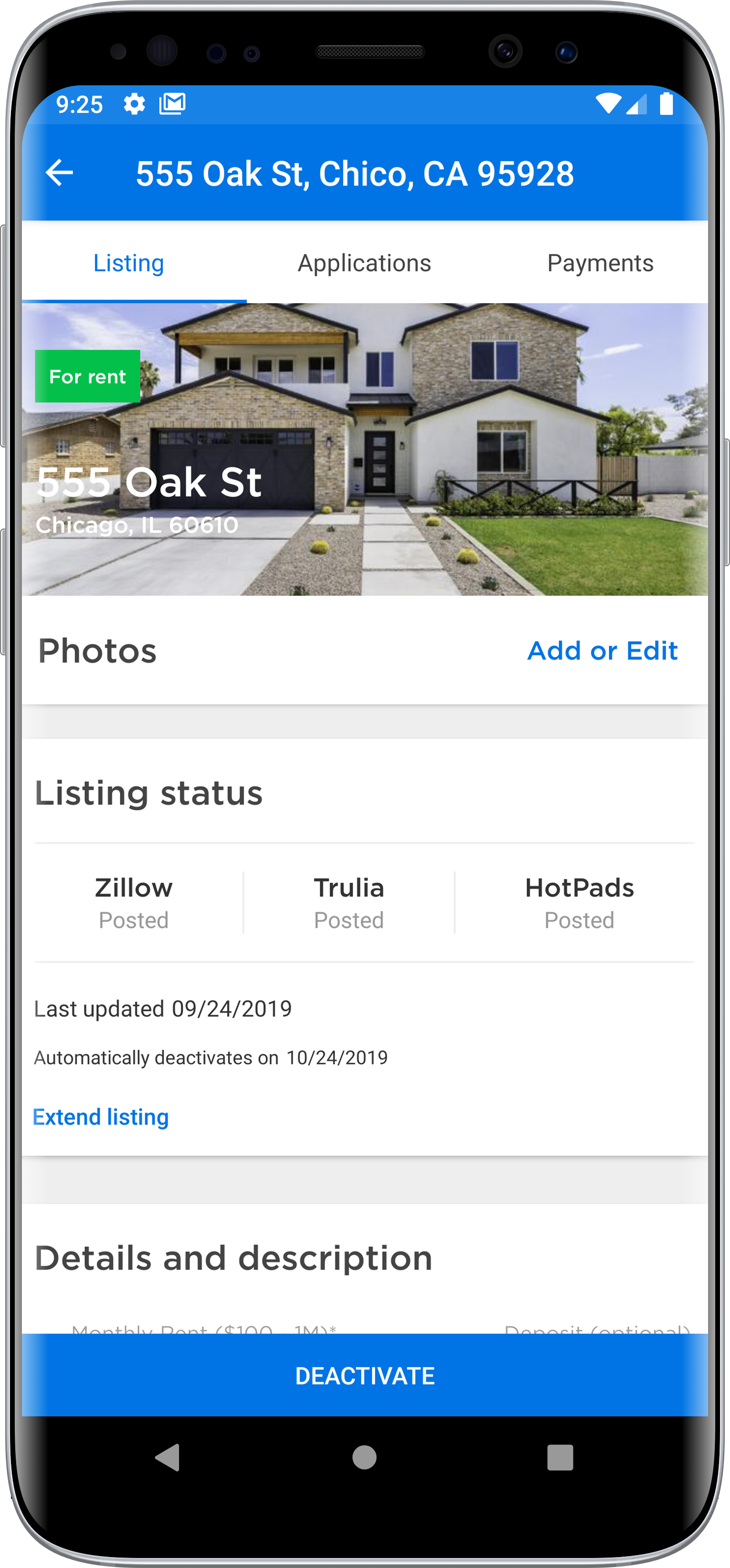This screenshot appears to be taken from an iPhone, evident by its thin silver edge, with two slim buttons on the left side and one on the right. The screen displays the time as 9:25. At the top, icons for Settings, Gmail, internet, and a fully charged battery are visible.

Beneath these, an address is displayed: "555 Oak Street, Chico, California 95928," alongside a left-pointing arrow. Below this are three categorized tabs: "Listing" (currently highlighted), "Applications," and "Payments." 

Within the "Listing" tab, there's a photo of a brick duplex with white walls and a brown garage door, accompanied by a cement driveway, a rocky area flanking the sidewalk, and a grassy section to the right. The listing specifies that the property is available for rent at "555 Oak Street, Chicago, Illinois 60610," indicating a discrepancy in the city and zip code from the earlier address. 

Further details include options for "Photos," "Add or Edit," and "Listing Status," with notes that the listing has been posted on Zillow, Trulia, and Hotpads. The last update was made on 09/24/2019, and the listing is set to automatically deactivate on 10/24/2019. The bottom of the screen features a blue bar labeled "Deactivate."